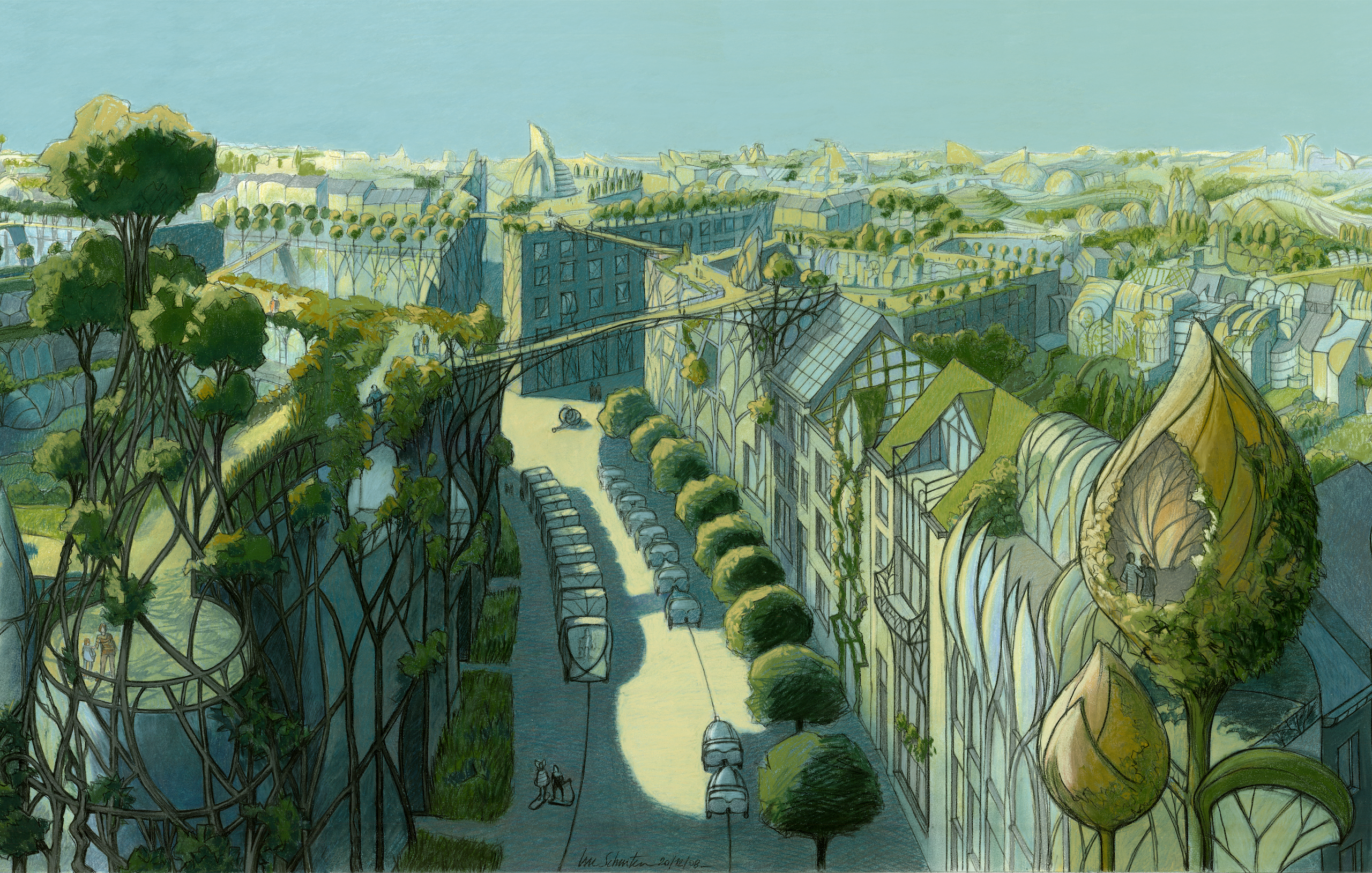This detailed illustration depicts a futuristic, utopian city crafted in a modern, possibly digital, artistic style. The cityscape showcases buildings intertwined with lush greenery, including trees, vines, and grass sprouting from rooftops and balconies. A prominent feature is the network of bridges and elevated walkways that connect various buildings, contributing to the layered, multi-dimensional architecture. On the left side, the building teems with the most vegetation, with branches forming footbridges to adjacent structures. Below, a street lined with uniform small cars, possibly on rails, is bordered by green trees and dotted with pedestrians. In the distance, whimsical giant snails can be seen, adding an imaginative touch. The overall setting under a clear blue sky highlights a harmonious integration of nature and urban living, complete with people inhabiting tree houses and platforms nestled within the green canopy.